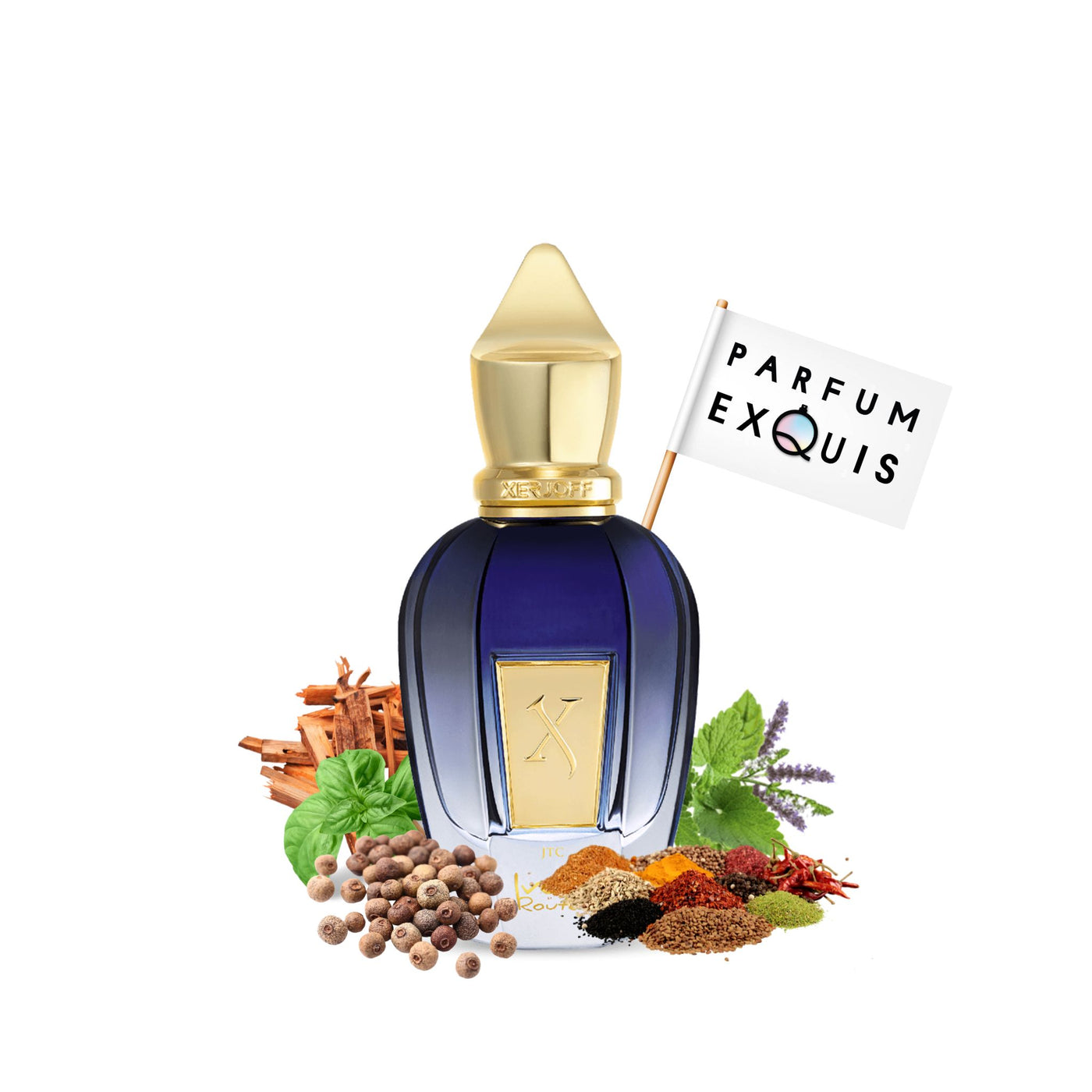This image features a sophisticated bottle of perfume named "Parfum Exquis." The bottle is crafted from blue glass adorned with curving ridges that add an elegant texture. It has a distinctive gold cap that resembles a Pope's hat, with an engraving of the name "Zernoff" along its edge. Attached to the bottle by a wooden stick is a small white flag bearing the name "Parfum Exquis." A prominent gold rectangle with an X logo graces the center of the bottle. The background is a stark, clean white, accentuating the array of colorful spices, herbs, and perhaps flowers surrounding the bottle. These items appear in various forms, including raw, powdered, and possibly wood chips, contributing to the sophisticated and exotic ambiance of the fragrance presentation.